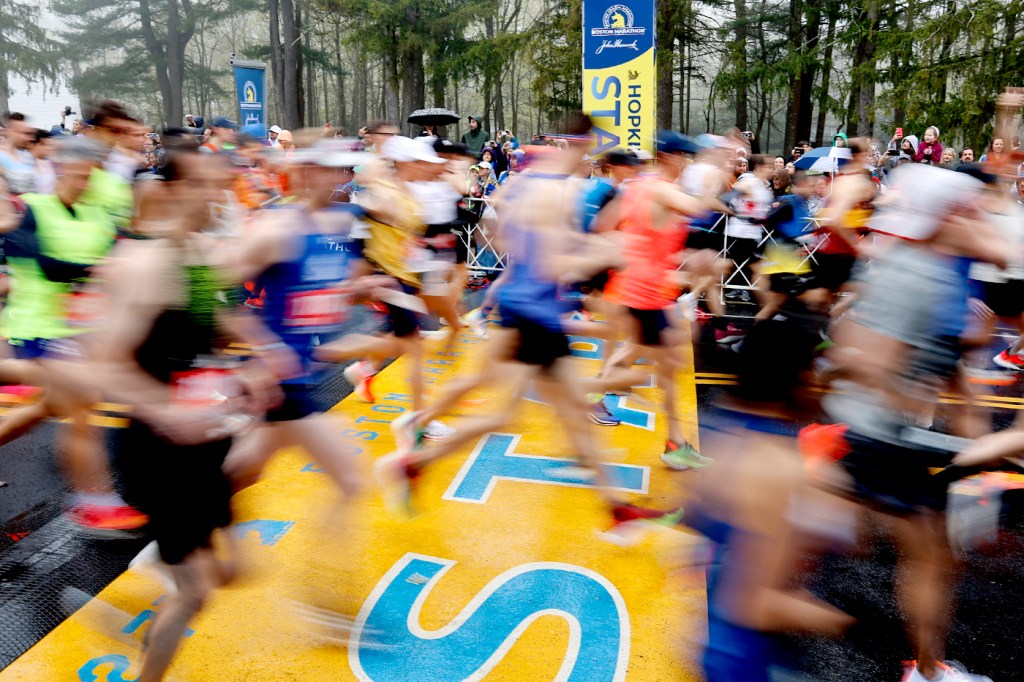This is a color photograph capturing the bustling start of the Boston Marathon. A large crowd of runners is crossing the prominently marked yellow start line with the word "START" in bold blue text. The scene is blurred due to their rapid motion, conveying a sense of speed and excitement. The background features a banner emblazoned with "John Hancock" and "Hopkinton," solidifying that this is the starting point of the famous race. Behind the runners, a white fence lines the pathway, with spectators gathered to cheer them on, some holding umbrellas, suggesting rainy weather. Tall trees and a misty, gray sky add to the overcast ambiance of the day. The majority of runners are dressed in shorts, short-sleeved shirts, and hats, undeterred by the damp conditions as they charge ahead.